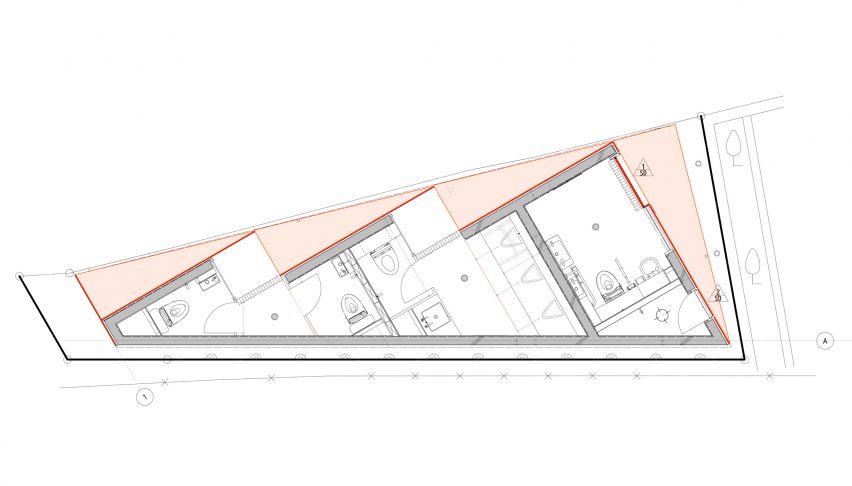This detailed blueprint showcases the corner section of a building, hinting at a triangular, rectangular structure with pronounced diagonal elements, reminiscent of mountain peaks. The building spans three distinct protrusions across the lot, each featuring pointed ends.

Highlighted in pink, areas likely representing grass or sidewalks surround the structure, complete with an area denoted by the letter "A," possibly significant for building semantics or planning sections.

Inside, the blueprint reveals multiple rooms, predominantly bathroom areas, evidenced by door openings and a variety of fixtures. The right section illustrates a multi-bathroom setup, with clear demarcations for toilets, sinks, urinals, and bath stalls. Black outlines and numerous thin lines suggest structural walls and divisions within the building. The entire diagram uses a peach color scheme, indicating different zones and is likely created using specialized computer software for architectural design.